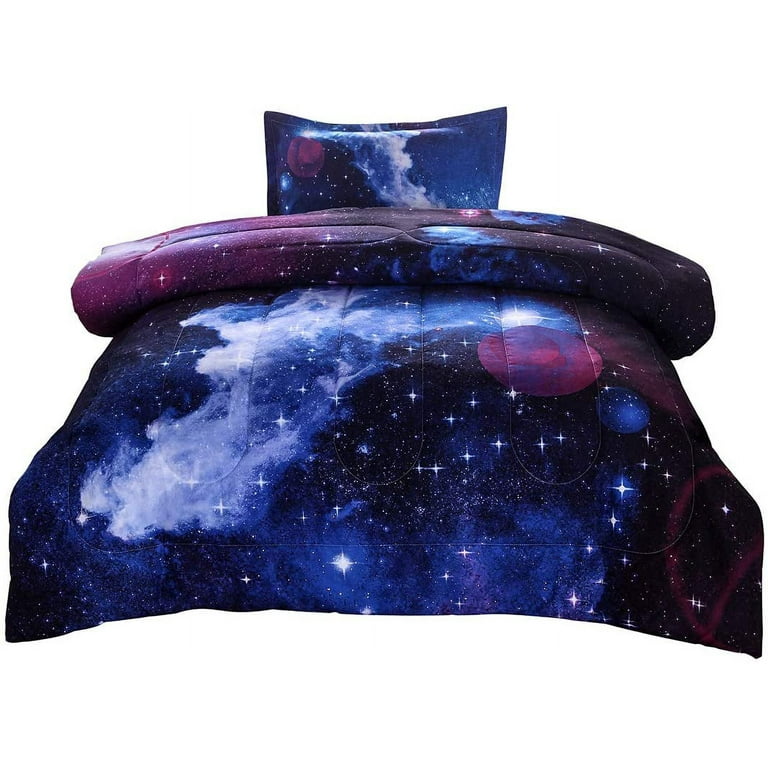The image presents a top-down view of a bed with a bed cover and pillow, resembling the appearance of looking into a glass jar or vase from above. The bed cover and pillow are intricately designed with an outer space theme, featuring a dark background adorned with deep blues, light blues, whites, and purplish pinks that beautifully depict stars, constellations, and galaxies. The coverlet spreads out expansively, showcasing a dramatic scene on a canvas-like white background devoid of visible borders. Detailed intricacies decorate the image, such as nebulae and gas clouds drifting to the left. The bed cover appears to fold slightly near the pillow, adding a touch of realism. The dark hues mixed with purple, deep blue-to-black accents, and a contrasting light gray create a visual effect reminiscent of a deep sky telescope view, evoking a sense of gazing into the night sky. Amidst this cosmic spread, there is also the subtle inclusion of a reddish planetary object. The ensemble is both meticulously crafted and celestial, capturing the infinite expanse of the universe on a cozy bedding set.